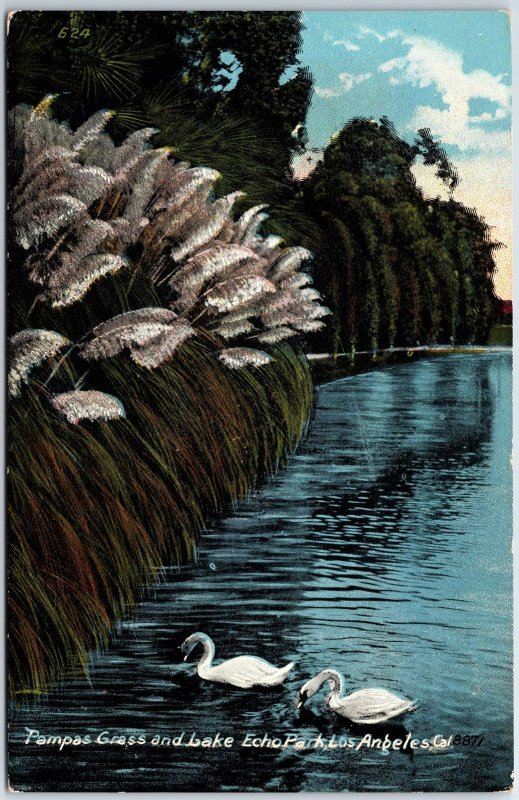This is an older painting, with slightly worn edges, depicting a serene outdoor scene at Lake Echo Park, Los Angeles, California. The composition is in a tall, portrait mode, capturing a tranquil lake that stretches from the bottom left to the middle right of the image. The water is painted in a rich, teal blue, accented by the sparkling highlights that suggest the play of light from the sky above. Two white swans grace the scene, one appearing to drink from the lake, adding a touch of life to the peaceful waters.

In the background, there's a lush display of pampas grass, detailed with brown and white tufts, cascading gently over the lake's edge. Behind the grass, a variety of trees rise, their green foliage punctuated by splotches of brown and white, giving the impression of layered depth and texture. Further back, more trees line the distant shoreline, adding to the scene's natural beauty.

The sky above is a vibrant blue, dotted with fluffy white clouds, which transition to a yellow-white hue near the horizon, suggesting the presence of sunlight. The painting's caption, written in white at the bottom, reads "Pompous Grass and Lake Echo Park, Los Angeles, California," with the number 8871 also inscribed below.

Overall, this detailed and enchanting artwork captures the tranquil beauty of Echo Park, rendered in a timeless style that evokes a sense of peace and natural splendor.